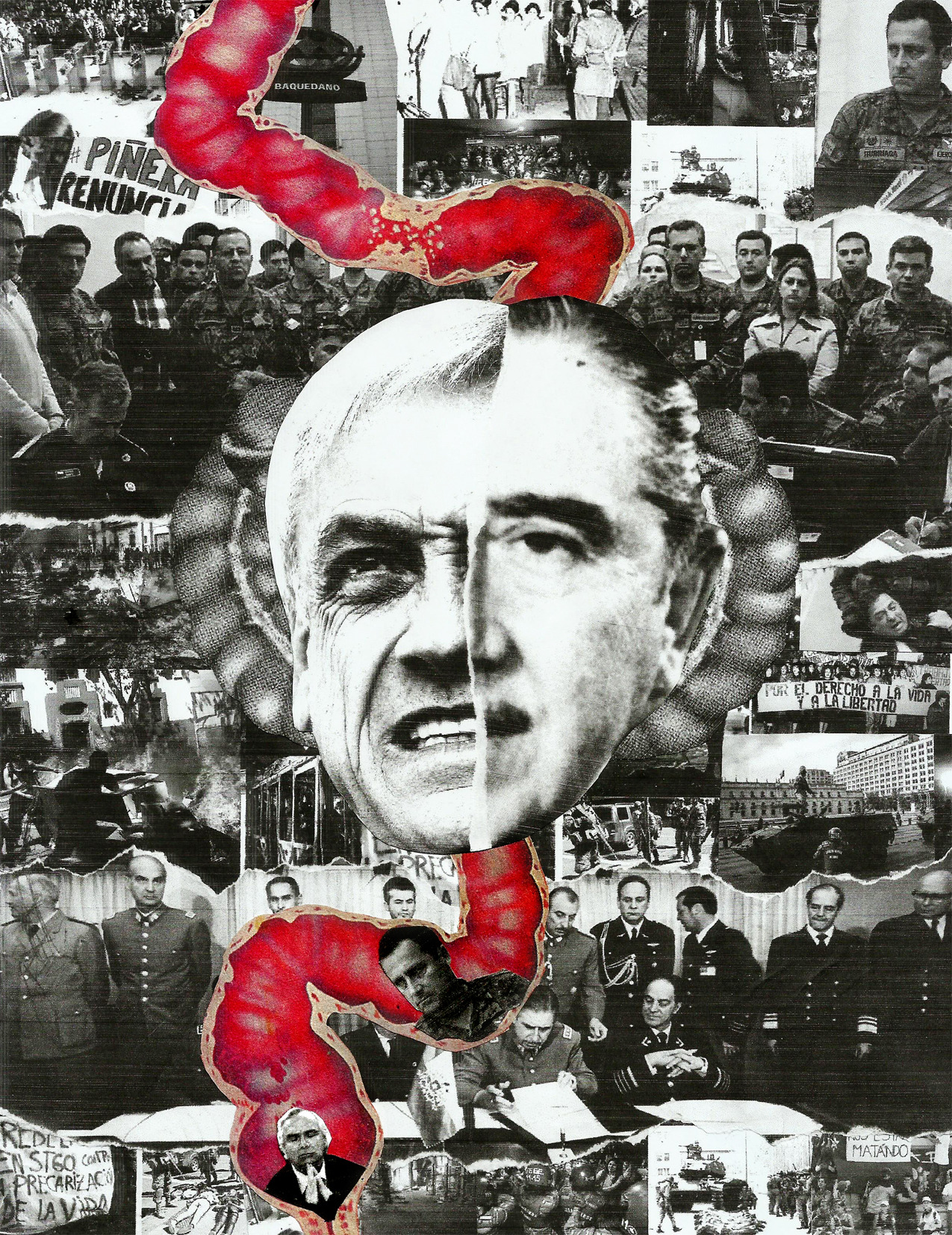The image is that of a highly elaborate and striking political poster, prominently featuring a collage of various black and white photos. Central to the poster is a large, black and white image of a man's face, seemingly ripped from a magazine, with another man’s face partially peeled away and hidden behind it. Surrounding this central face, extending from both the top and bottom, are reddish anatomical tubes designed to resemble intestines, imparting a visceral and provocative message. Within these intestines, other political figures appear, some positioned as if they are to be expelled from the colon. At the base of the image, there are several people in military attire; one of the uniforms appears to be Nazi, suggesting a historical or authoritarian connotation. The wider collage integrates diverse elements, including photographs of activists, protest signs, and military machinery such as tanks, interspersed throughout the scene. The poster appears to be in a language that may be Spanish or Portuguese, adding a layer of cultural and political context that is non-Anglophone. The color palette is mainly black, white, gray, red, and some brown tones, emphasizing the stark and somber tone of the artwork. This poster is a deeply political piece, possibly considered outsider art, combining graphic and provocative elements to convey its message.